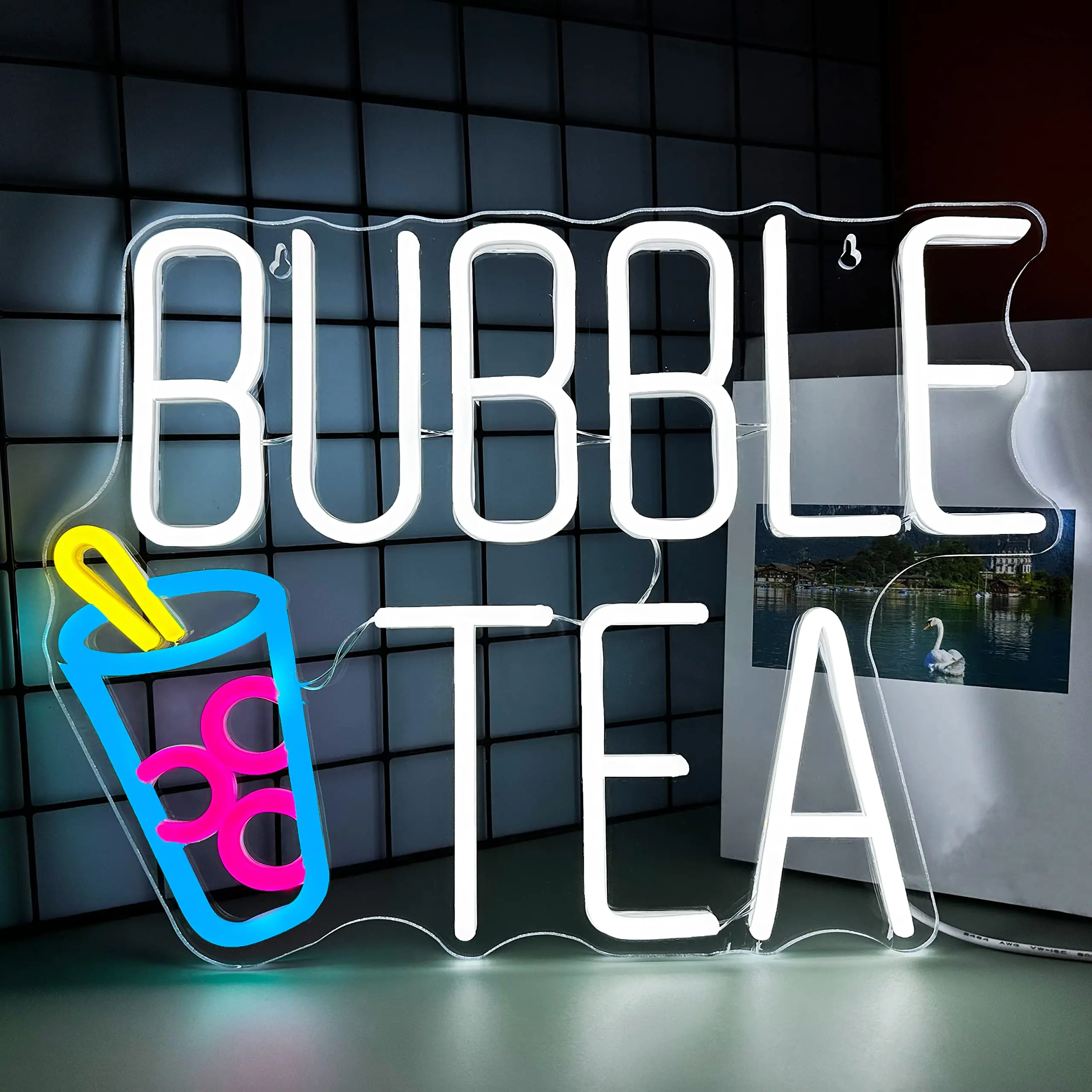This image features a prominently displayed fake neon sign that appears to be LED-lit. The sign, which occupies about 80% of the foreground, is crafted into a piece of plexiglass. Routed grooves are filled with LEDs and painted in their respective colors to simulate neon tubing. The sign reads "bubble T" in white text, with "bubble" positioned above "T." To the left of the letter "T" is an artistic rendering of a boba tea cup. This cup is outlined in blue, filled with three purple rings representing tapioca pearls, and topped with a yellow spoon sticking out from its lid. Visible wires connect the letters, hinting at how it is illuminated. The background consists of a gray wall with a black crosshatch pattern and another wall to the right, which is either white or light gray. This secondary wall features an outdoor scene depicting a swan on a lake alongside a house, possibly a picture or a television screen. The floor beneath the sign is medium gray concrete.